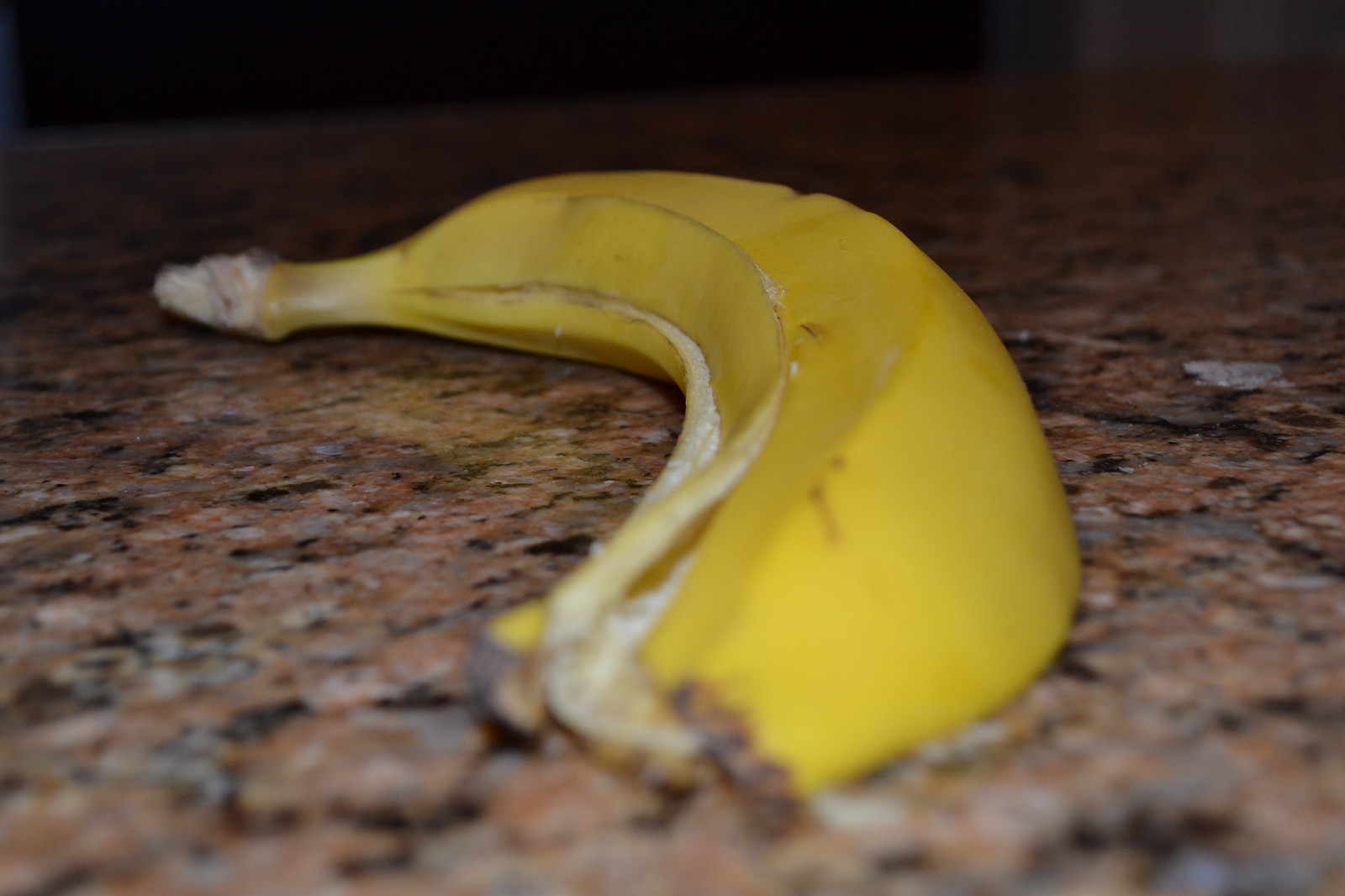A detailed caption for the image could be:

"Centered on a stone countertop, a discarded banana peel, its bright yellow hue marred by small black markings, lays prominently in the foreground. The peel is void of the banana, showcasing a smooth surface with no significant bruises. The stone countertop beneath it features an intricate mosaic of colors, including blacks, whites, light blues, browns, tans, and creams, likely indicating a granite material. Towards the upper right, the background fades into dark colors, perhaps a deep blue or black, creating a stark contrast that highlights the vibrant banana peel. The countertop dominates about 90% of the image, accentuating its speckled pattern and providing a detailed, textured backdrop to the solitary banana peel."